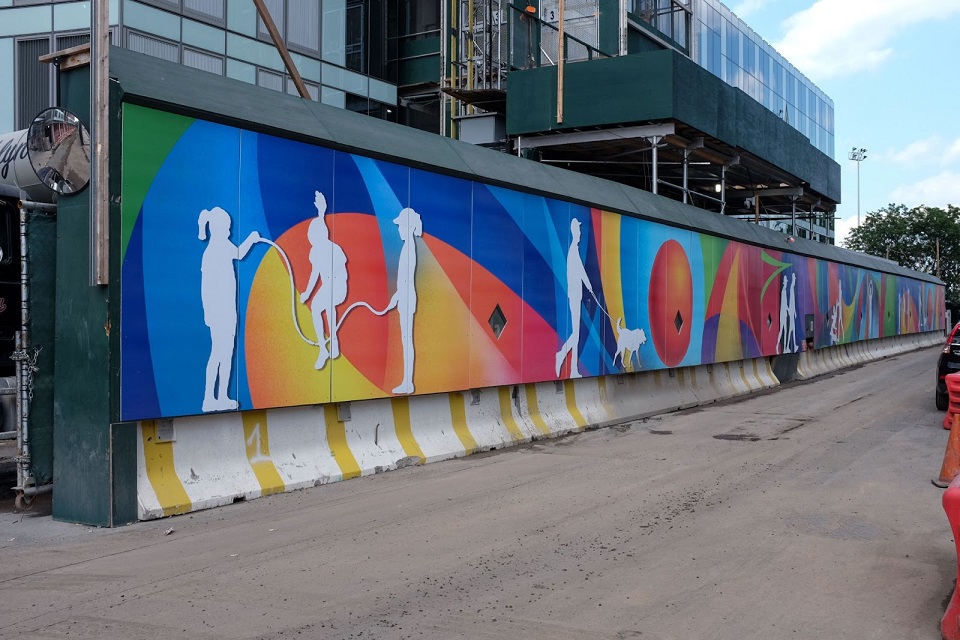In this vivid urban scene, a long, colorful mural adorns a wall that stretches across a city street, positioned in front of a large glass building with visible scaffolding and windows. The decorative wall, spanning from the left middle to the right middle of the image, features an array of bright colors including orange, yellow, red, white, blue, light blue, green, black, gray, forest green, and sky blue. The mural depicts a series of white-outlined figures on different panels: two children playing with a jump rope, a person with a dog, a couple walking, and another person walking with a child, with a backdrop of abstract colored shapes resembling beach balls in various hues. At the far left, a large mirror is mounted above the cement curb beneath the panels, allowing visibility down the road, which is lined by the wall and the gated entrance. Sky partially visible in the top right corner completes the vibrant and bustling cityscape.